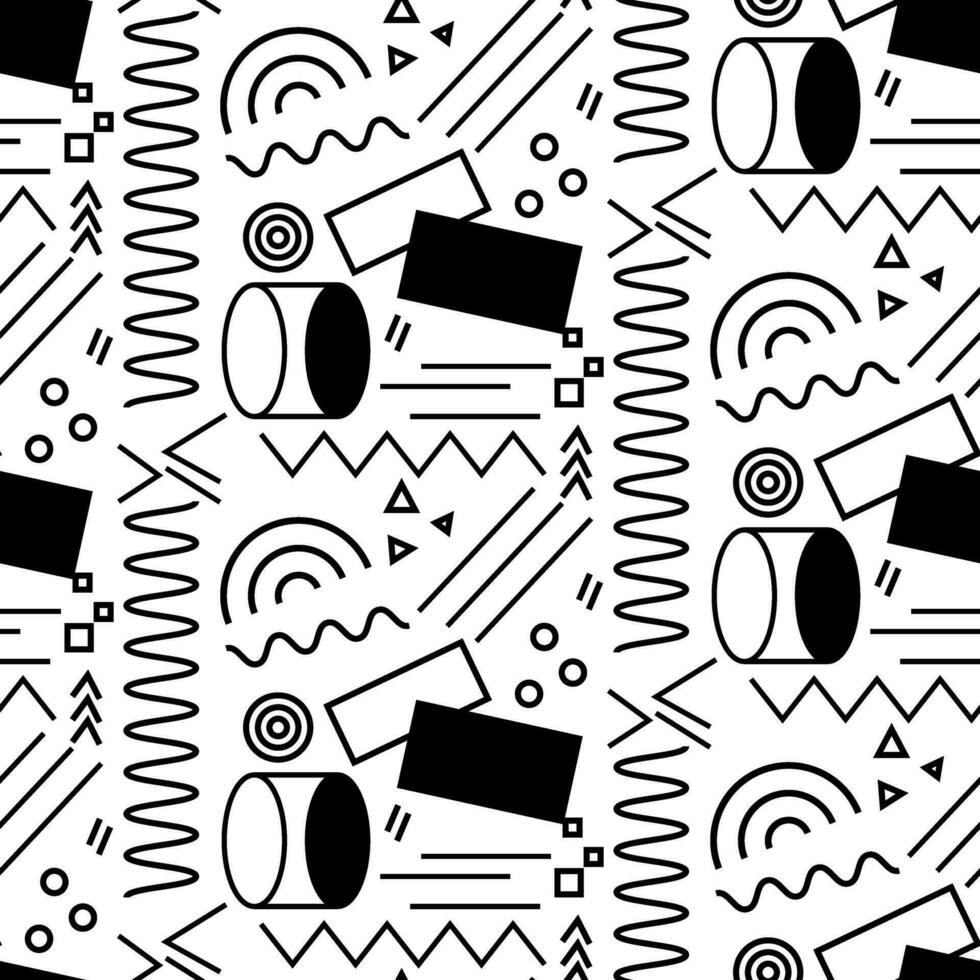This black and white image exudes a modern art aesthetic with a strong 90s vibe. It features a captivating assortment of geometric shapes arranged in a repetitive pattern that spans both vertically and horizontally. You can see a variety of squiggly and wavy lines, zigzags, and V-shapes interspersed with different forms like triangles, squares, circles, and half-circles. Notable for its high contrast, the design includes concentric circles and half-circles that add depth to the overall composition. Cylinders are depicted with both black and white oval tops, and rectangles are either outlined or fully filled in black. Additionally, there are sections of the image that resemble targets, while arrows point upwards, enhancing the dynamic feel of the scene. Elements like rhombus-like shapes—possibly just rectangles with cut-off corners—add to the complexity. The entire arrangement of these black shapes against a white background creates a visually striking and intricate wallpaper-like pattern that invites the eye to explore its repeating motifs and designs.